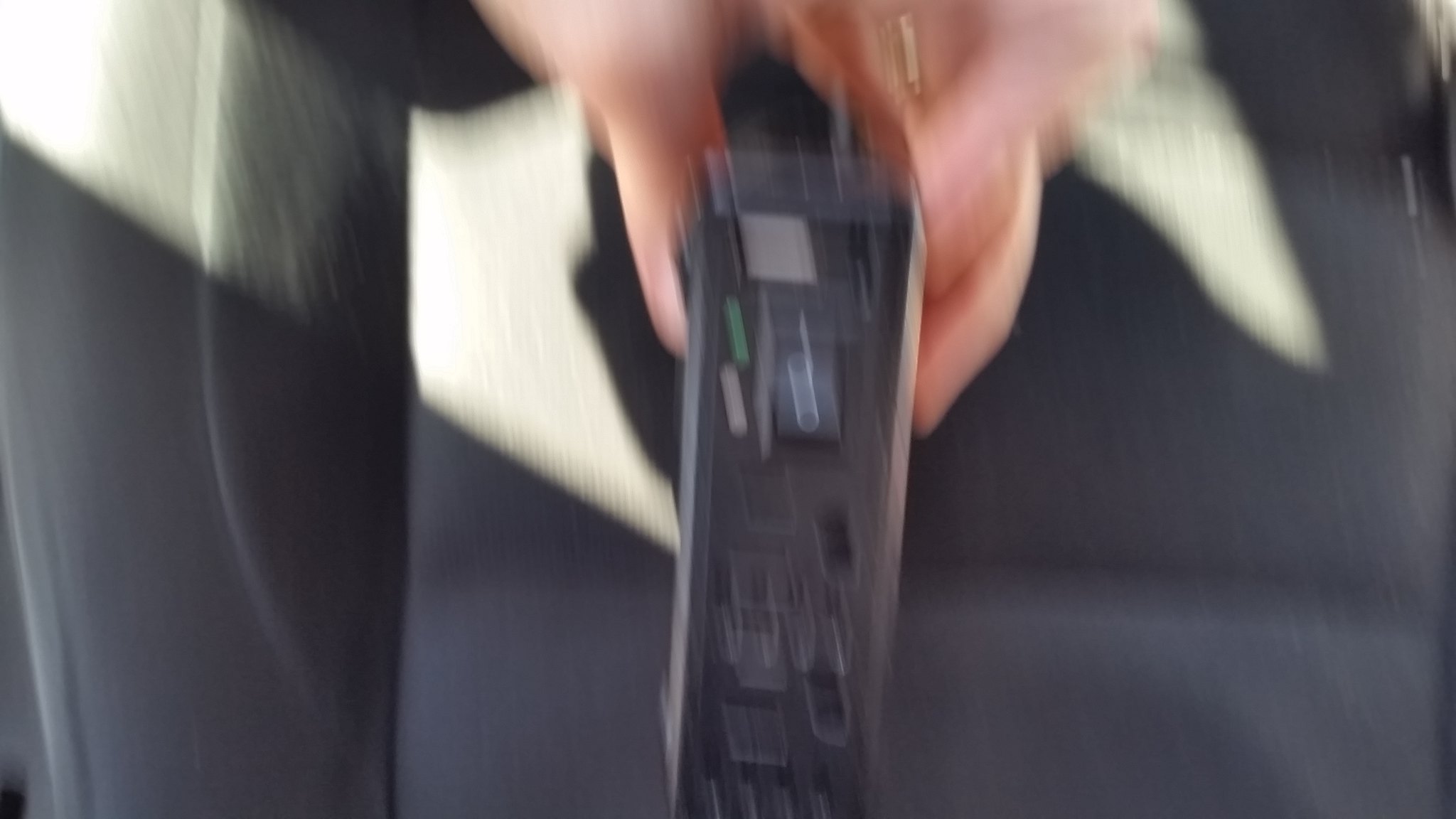The photograph depicts a person's hand holding a black control device in the center of the frame. The image is very blurry, likely due to motion, creating a doubled effect where details are hard to distinguish. The background appears predominantly black, suggesting it might have been taken inside a car, with the seat partially visible. The control in the hand has an identifiable power button, but the entire scene is difficult to interpret clearly due to the significant blurriness. The photograph seems to capture a quick, motion-filled moment, adding to the overall unclear nature of the objects and background.